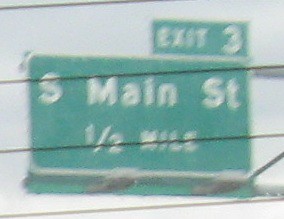The image depicts a street sign viewed through the windscreen of a car, slightly blurred. The sign is green with white text and is bordered in silver. At the top right corner, there's a smaller rectangular sign that says "Exit 3" in white letters on a green background. Below it, the larger main sign reads "S Main St" and "1/2 mile." Four black lines, possibly from a lattice or some obstruction, run across the image. The scene is set against a cloudy grey sky, and the road lines are faintly visible beneath, enhancing the sense of viewing from within a moving vehicle. A part of the pole supporting the sign is visible to the right.